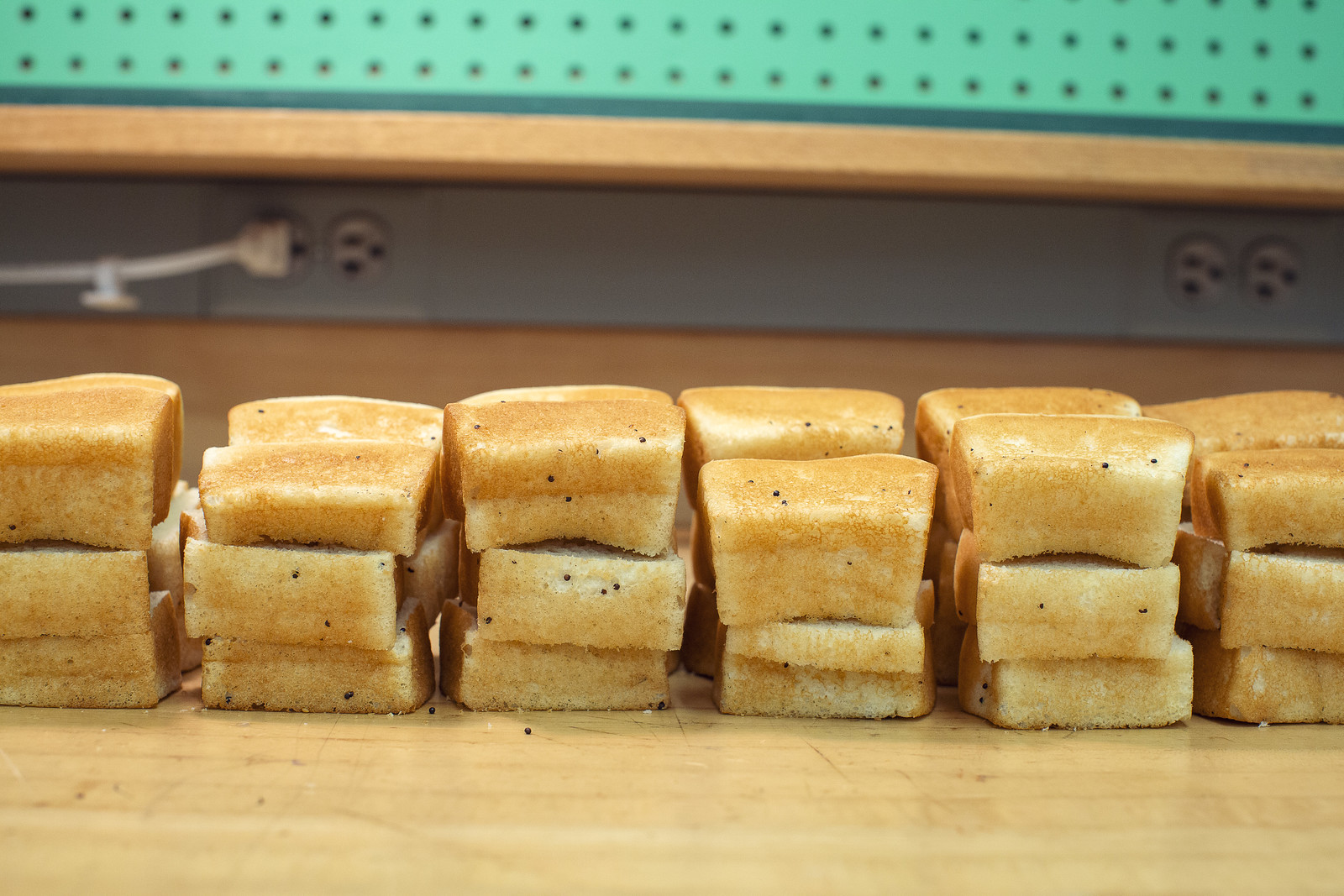The photograph is a horizontally oriented color image, bathed in a warm honey brown tone. It portrays a line or stack of golden brown, spongy-textured pieces, possibly bread or spongy cake, adorned with black specks that resemble poppy seeds. These pieces stretch from the left to the right across a wooden cutting board or shelf in the mid-ground. The background showcases a strip of metal with wall sockets, one of which is occupied by a white plug, interrupting the predominantly light backdrop. Above this metal strip, a green pegboard stretches across the top portion of the image, featuring evenly spaced black holes. The entire setup suggests a homely or production-oriented environment, likely for making or displaying these bread pieces.